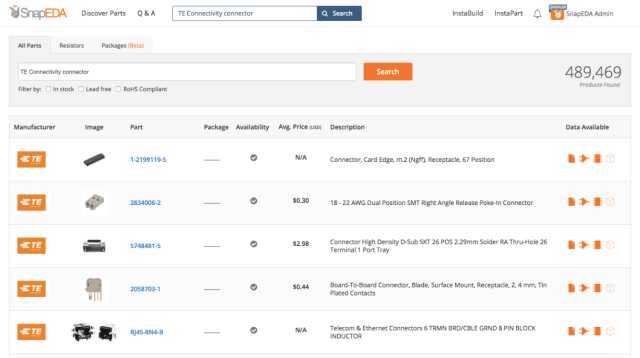The image showcases a comprehensive screenshot of an electronic component search on the SnapEDA website. Set against a white background, the top section features the SnapEDA logo on the left, with navigation links labeled "Discover Parts" and "Q&A," followed by a prominent search bar. The search bar allows users to input keywords to find specific electronic parts, and is accompanied by an orange search button. Just below this search interface, a notification indicates that 489,469 results have been found.

The results are organized in a detailed table format, featuring several columns: "Manufacturer," "Image," "Part," "Package," "Availability," "Average Price," "Description," and "Data Available." Each "Manufacturer" entry displays an orange box with the initials “TE” inside it. The "Image" column contains visual thumbnails of the respective components. The "Part" numbers are highlighted in blue text, making them easily identifiable. All listed items in the "Availability" column are marked with check marks, indicating they are in stock. Additional columns provide detailed information about the parts, including pricing and brief descriptions.

This well-structured layout ensures that users can efficiently locate and identify necessary electronic components with ease, making SnapEDA a valuable resource for engineers and hobbyists alike.